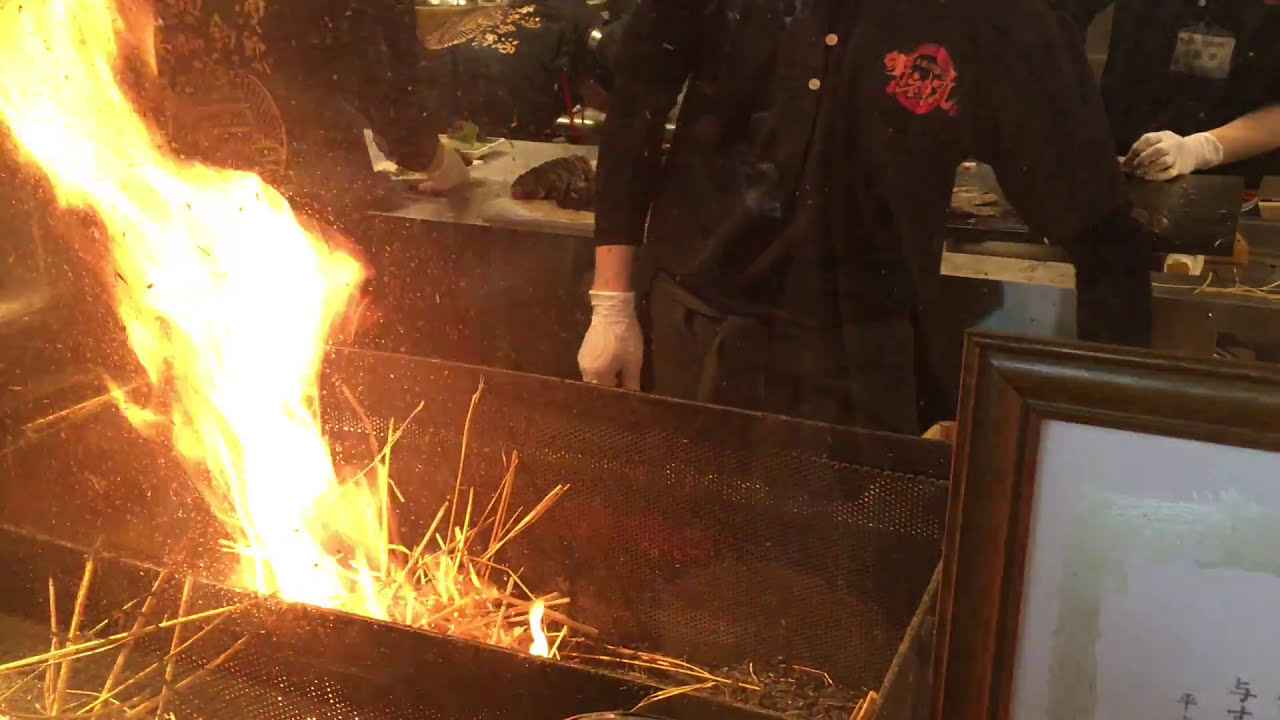The image depicts a striking and somewhat enigmatic scene mainly centered around a vigorous fire contained within a sizable metallic bin or receptacle. The flames are fueled by what appears to be straw or hay, reaching dramatically towards the top edge of the image. Just behind the fiery spectacle stands a man clad entirely in black, identifiable by his black button shirt featuring a red logo on the left side. He is also wearing transparent white rubber gloves on his right hand, suggesting he is engaged in food preparation. To the right and left of the image, partially obscured by the flames, additional individuals can be discerned, all similarly attired in black outfits with rubber gloves. Behind these figures, there's a counter where more people are busy preparing food, possibly handling meat. The overall scene suggests a busy, dynamic environment that could be interpreted as a professional kitchen setting, perhaps in a restaurant or a hibachi-style grill, underscored by the presence of a framed picture partially visible to the right of the main subject.